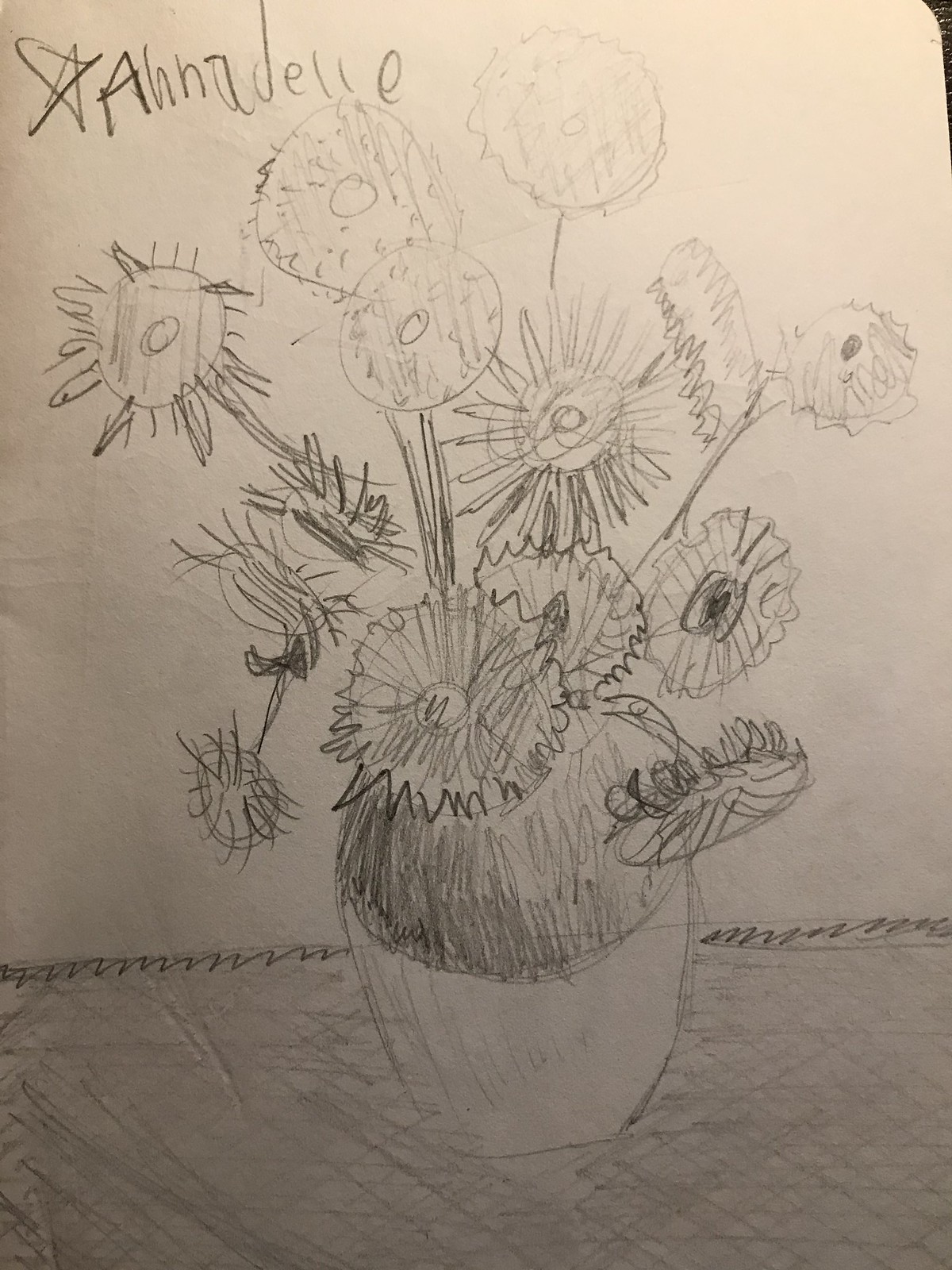This intricately detailed pencil sketch depicts a scene featuring a vase filled with several flowers that resemble sunflowers. The vase, set on a table, is outlined in pencil with a white cloth draped over the surface, adding depth and texture to the composition. Emerging from what appears to be a layer of dirt within the vase, the flowers display varied petal structures, contributing to the charm of the artwork. In the upper left-hand corner, a star accompanies the artist's signature, 'Annadelle,' clearly indicating the creator's personal touch. The entire piece, drawn carefully on white paper, captures an attempt at rendering sunflowers, showcasing the artist’s attention to detail and commitment to their craft.